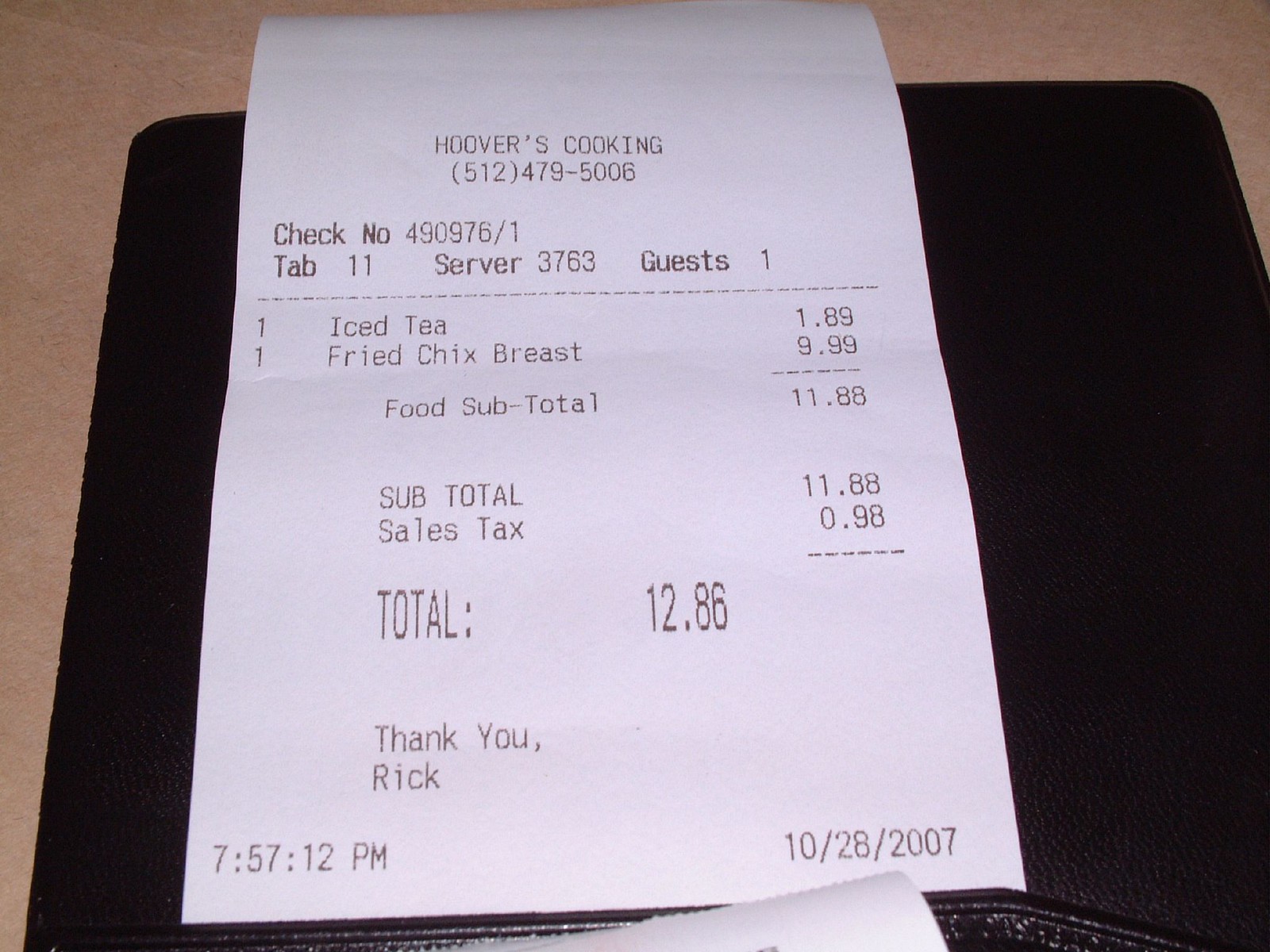A detailed caption:

"A detailed restaurant receipt is prominently displayed against a layered background. The receipt, which is the central focus of the image, sits atop a black surface resembling a mouse pad, and this black background is itself placed on a tan surface. The white receipt is printed with dark lettering and features the branding 'Hoover's Cooking' along with a contact phone number. In an organized list format, the receipt documents various transaction details: check number, tab number, table number, server number, and the number of guests. The items ordered include an iced tea and a fried chicken breast, amounting to a subtotal of $11.88 before tax and a total amount of $12.86 paid. The server's name is identified as Rick, indicated by the phrase 'Thank you Rick' on the lower left corner. The receipt also includes a timestamp and a date, specifically October 28, 2007, located in the lower right corner."